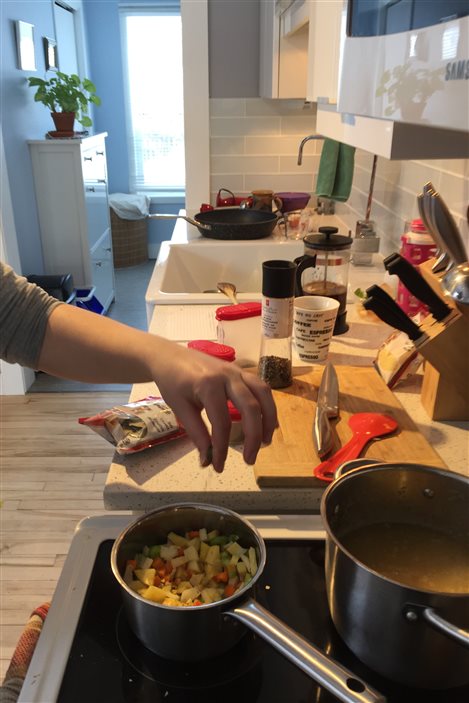In this vibrant color photograph taken in a kitchen, a left hand protrudes from the left side of the frame, actively engaged in the culinary setting. At the bottom, a black stovetop takes center stage, hosting two pots in the midst of meal preparation. Moving rightward, a butcher block cutting board is prominently positioned, accompanied by a sleek, silver knife lying beside a red spatula. The upper right corner reveals another cutting board, adjacent to a butcher block style knife holder, adding to the kitchen's organized atmosphere. Beyond this, a pristine white sink gleams, reflecting the well-maintained space. In the upper left corner, the image extends into another room characterized by blue walls and a window adorned with blinds. A small, narrow dresser stands to the left, decorated with a lush green houseplant and a terracotta bowl, enhancing the homely ambiance.